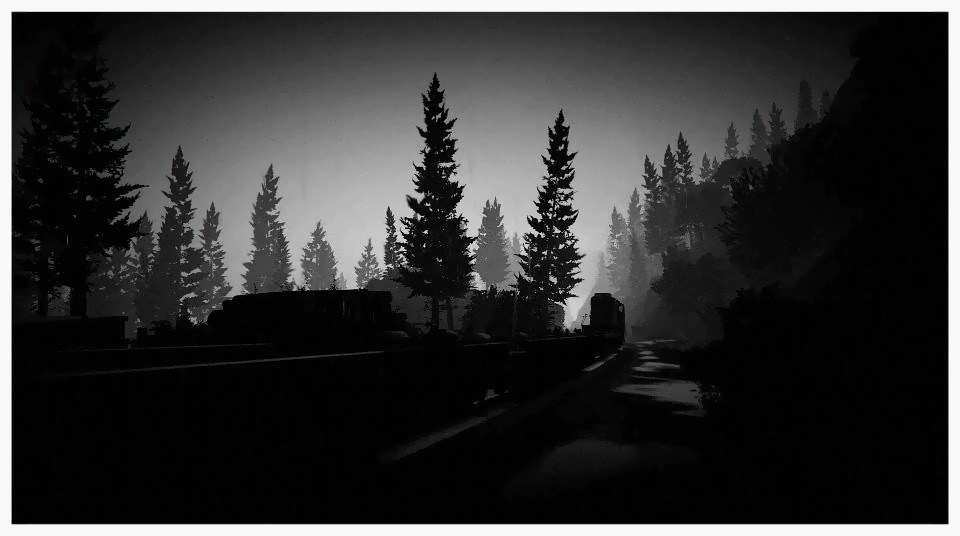A vivid, potentially computer-generated night-time scene reminiscent of a video game environment. The bottom of the image features stark black areas on both the left and right ends. On the right, the dark silhouette of trees creates a dense background, contrasting with the left side where a prominent structure, possibly part of a bridge, comes into view. A road, intermittently illuminated in shades of light gray, splits the scene, with the rest cloaked in deep shadows. Moving along the road towards the back of the image is a long, black vehicle that resembles a train. The backdrop is peppered with more dark trees against a sky that transitions to a light gray tone, emphasizing the tranquil and mysterious ambiance of this night-time setting.